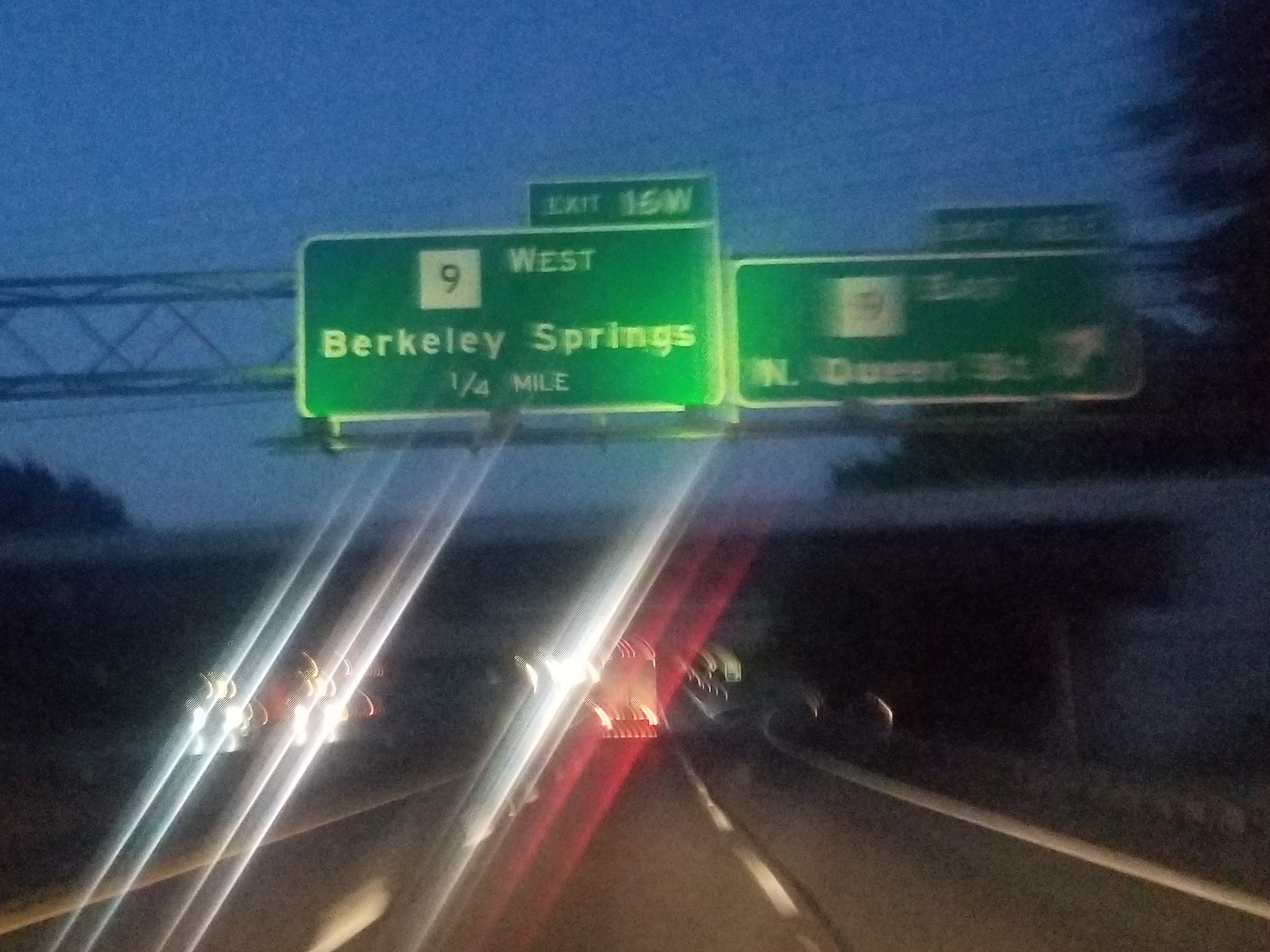The image depicts a nighttime scene on a multi-lane highway, viewed through the windshield of a moving vehicle, rendering the scene blurry. The dark blue night sky contrasts with the blurred streams of light from the headlights of oncoming traffic and the taillights of vehicles ahead. The highway, flanked by tall green trees on both sides, features a median separating the northbound and southbound lanes. Overhead, a large structure supports two prominent green traffic signs. One clearly reads "Exit 16W, 9 West, Berkeley Springs, 1/4 mile," while the other, partially obscured and blurred, appears to indicate "9 East" with a diagonal arrow pointing right and references North Queen Street. Further in the background, an overpass spans the highway, adding to the layered complexity of the scene.